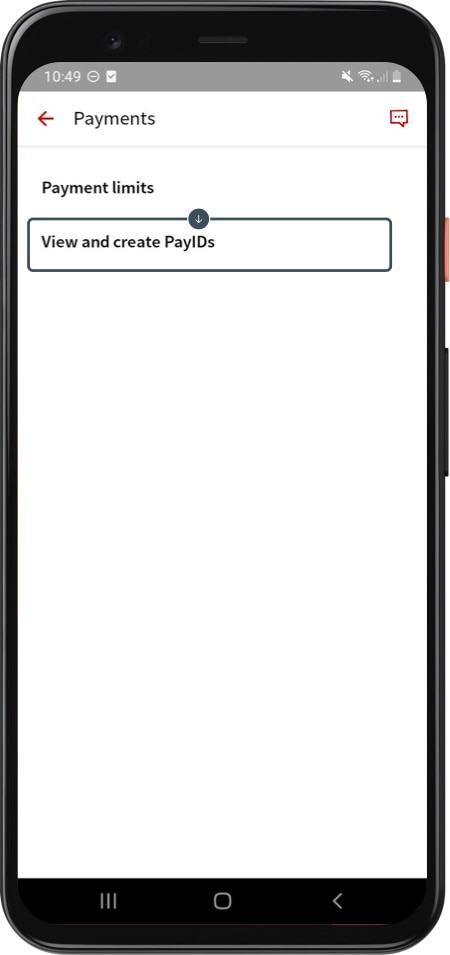The image depicts a payment screen on an iPhone, showcasing various screen elements and details: 

At the top, the status bar displays the connection icons, battery life indicator, and the time, which is 10:49. Below the status bar, the screen has a header that reads "Payments" in black, accompanied by a red left-pointing arrow and a red payment icon.

Under the header, there is a section titled "Payment Limits." This section contains a gray box with an 'i' within a circle and the text "View and create Pay IDs" written inside the box. The remainder of the screen is a blank white space, indicating that no Pay IDs have been created yet.

At the bottom black part of the phone screen, there are three vertical lines, possibly implying a menu button. Next to it is a square outlined in white with a left-pointing arrow, likely another navigation feature. These navigation elements suggest options for additional actions or accessing more information.